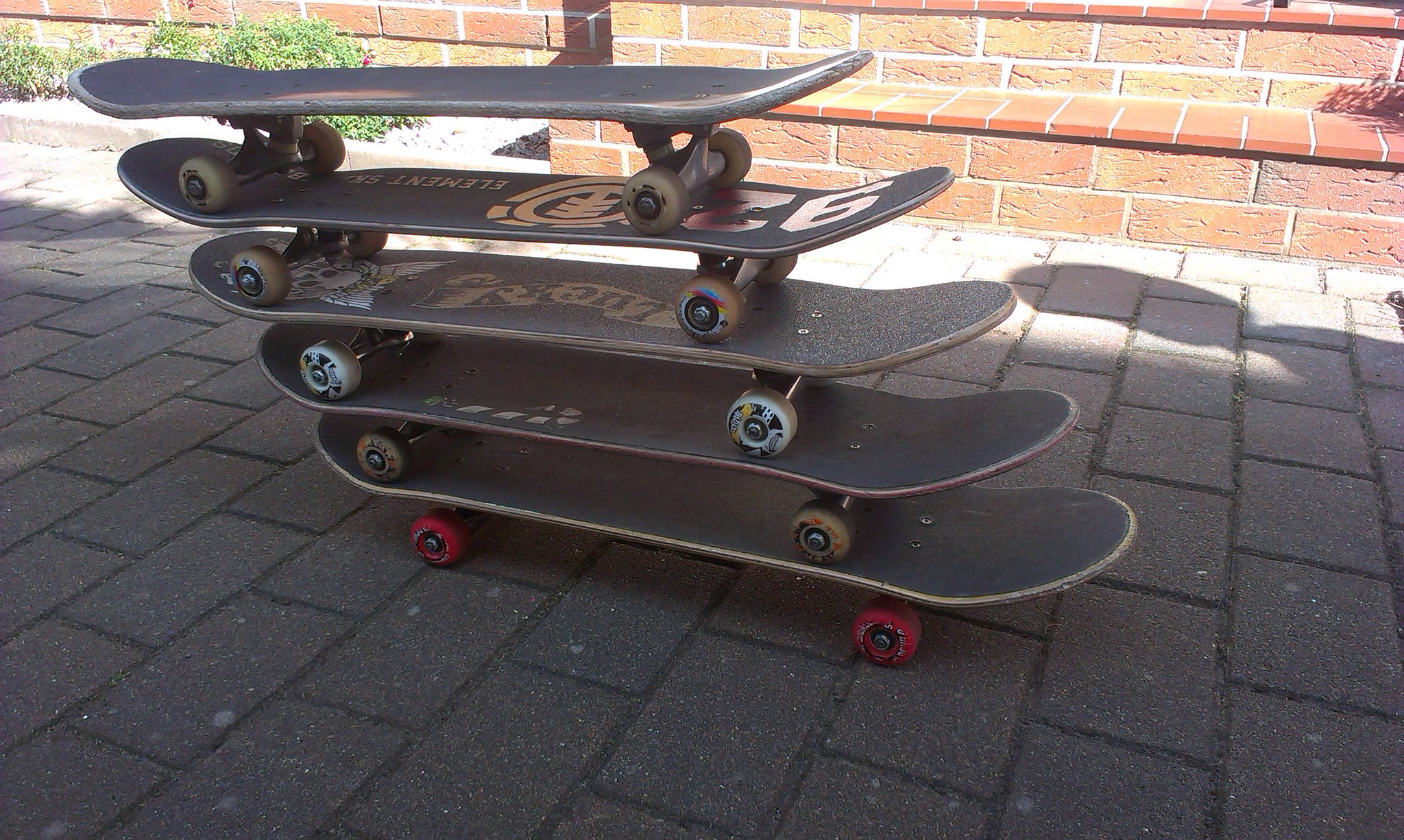This photo showcases a group of five skateboards stacked in a staggered formation on a gray tiled sidewalk. Each skateboard is predominantly black but distinguished by the color of its wheels. The skateboards are arranged so that each one on top is slightly set back from the one below it, creating a cascading effect from right to left. The bottom skateboard features red wheels, and as we move up, the wheel colors change to brown, silver, brown, and brown again. The staggered alignment creates a shadow, likely cast by the top skateboard, which is visible on the brick wall behind them. Also visible are the green grass and shrubbery to the left of the picture, adding a touch of color to the scene dominated by the gray sidewalk and brick background. The sunlight falls on the brick wall but leaves the sidewalk shaded, enhancing the details of the stacked skateboards.